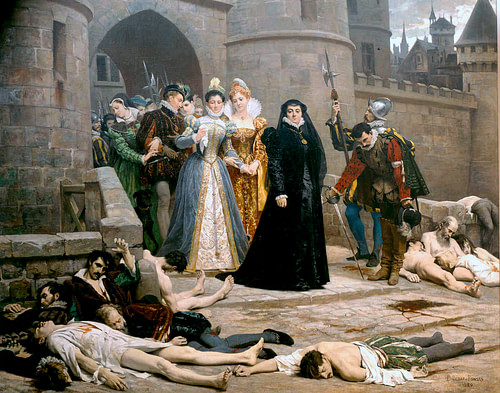This intricate painting captures a dramatic medieval Renaissance scene set within the confines of a grand castle. At the forefront, a group of elegantly dressed nobles, their colorful and luxurious garments signaling their high status, stands in stark contrast to the chaos before them. Prominently, a woman in a severe black dress and a man dressed in a distinguished white outfit lead the group. Flanking these nobles are two soldiers, one brandishing a pike with a steel helmet gleaming dimly in the muted earthly tones of the painting.

The nobles stand on a bridge with open gates behind them, their expressions detached as they survey the distressing scene in front. Scattered on the ground are bodies of several men, their modest attire—simple white shirts, many without pants—suggesting they are of a lower class. Blood stains the ground, and the disarray of their disheveled and partially stripped clothes implies they have recently been in a violent conflict.

The juxtaposition of the composed, untouched nobles against the grim backdrop of violence and death evokes a powerful narrative of social disparity and indifference, encapsulating a moment of historical intrigue and turmoil within the castle walls.